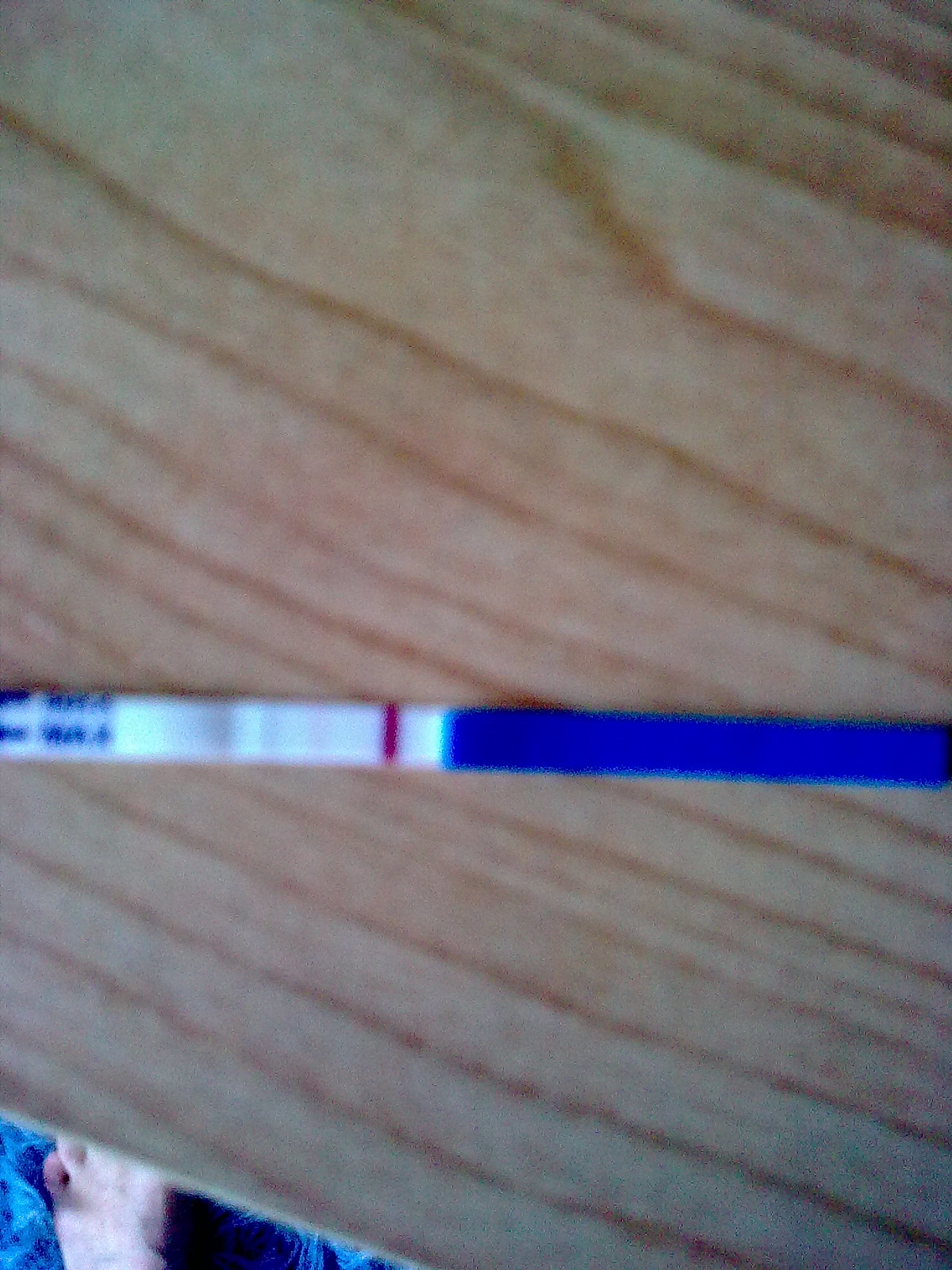A close-up photograph showcases a blurred beige fabric, featuring rows of darker brown lines that add texture to the material. Nestled on this fabric lies a small, intriguing strip that appears to be a testing device, potentially for chemical levels or a blood test. The strip is divided into two halves: the upper half is white, adorned with blue text and a distinctive red marking, while the lower half transitions into a solid blue. The overall lack of sharpness makes the finer details elusive, yet the colors and lines stand out, providing a subtle contrast against the neutral background of the fabric.